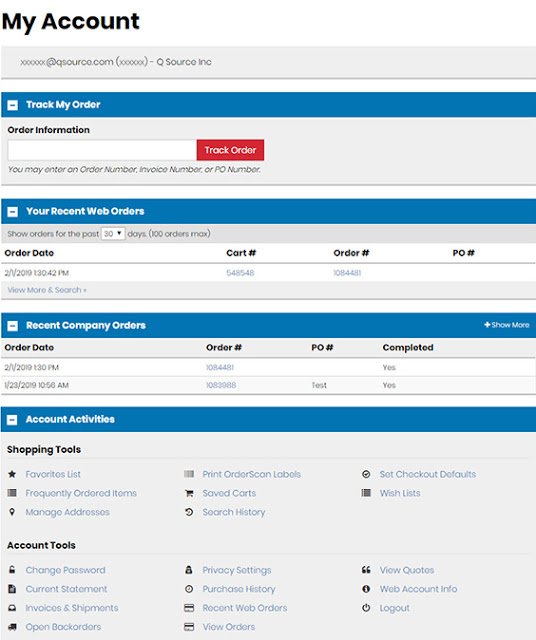In the image, a detailed overview of the user's account page on QSource.com is displayed. At the top, the account associated with the email "xxxxxx@qsource.com" is shown, labeled as "xxxxxx - QSource, Inc." There are various options available, including "Track My Order", "Order Information", and "Track Order". Users may enter an order number, invoice number, or PO number to track their orders.

The section titled "Your Recent Web Orders" allows users to display orders from the past 30 days, with a maximum of 100 orders. Specific order details are shown, such as:

- **Order Date:** February 1st, 2019
- **Cart Number:** 548548
- **Order Number:** 9084481

In the "Recent Company Orders" section, more orders are listed with detailed timestamps:

- **February 1st, 2019 at 1:30 PM**: Order 1084481
- **January 23rd, 2019 at 10:56 AM**: Order 1083988

Several account activities options are available, including "Shopping Shows", "Favorites List", "Frequently Ordered Items", "Manage Addresses", "Print Order", "Scan Labels", "Saved Cart", "Search History", and "Change Password". Additional features include access to current statements, invoices and shipments, open back orders, privacy settings, purchase history, recent web orders, viewing quotes, and web account information. Users can log in to manage their accounts and view pertinent details.